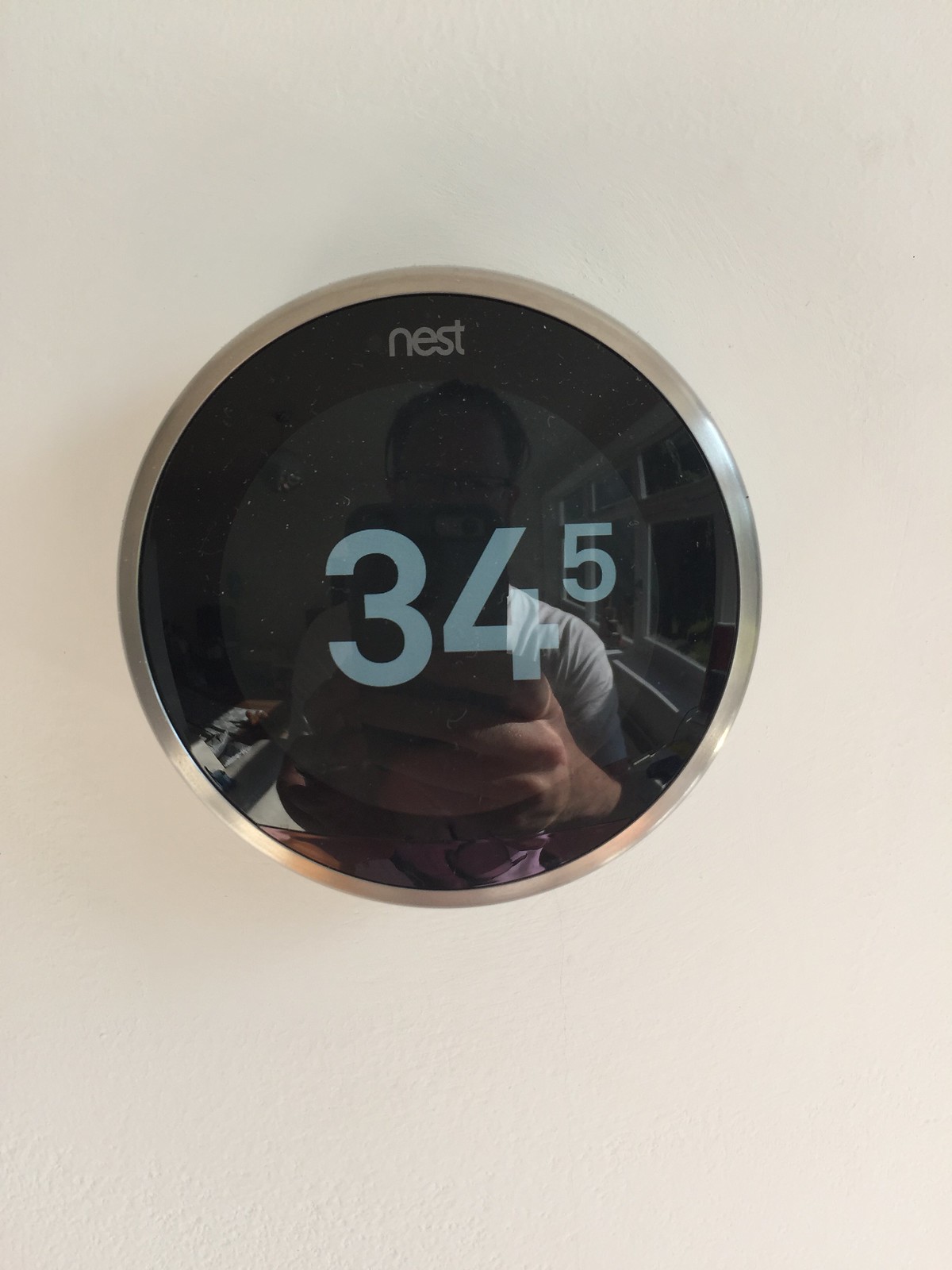The image depicts a Nest thermostat affixed to a white wall. Encircling the sleek, compact device is a silver ring, followed by a black outer circle, and an inner circle of a slightly lighter shade of black. Reflecting off the glossy surface of the thermostat, a middle-aged man with balding short hair and glasses is visible, holding up his smartphone to capture the shot. He is wearing a white t-shirt, and his hands are positioned in such a way that they obscure most of his face, only slightly revealing his nose.

Prominently displayed in the center screen of the thermostat is the number "34," with a smaller "5" positioned just above the "4." The reflection within the device reveals an interior scene, possibly a cozy living room, with bay windows that offer a view of a lush lawn outside. A couch adorned with pillows or blankets is partially visible, but the image is somewhat distorted because it is a reflection of a photograph within a photograph. The word "Nest" is elegantly printed at the top of the middle black circle on the device. The overall setting appears to be a comfortable home environment with white walls.